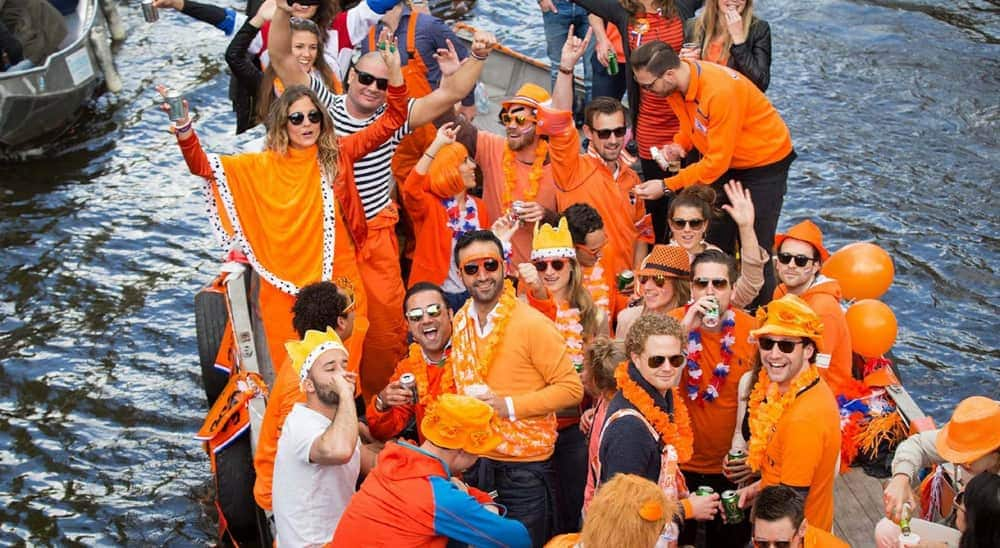This image captures a lively crowd of around 20 to 30 people packed onto a small barge or boat on the water. The crowd, appearing to celebrate, largely wears orange attire; many women and some men are clad in orange togas, while others don orange shirts, hats, and some orange caps or chaps. Scattered amongst the crowd are a few orange balloons, and most of the revelers sport sunglasses, shielding their eyes as they cheerfully look up at the camera with raised, outstretched arms. The scene exudes a festive atmosphere, with some drinking from cans, indicative of a party-like event. Amidst this sea of orange, two men stand out; one wears a white t-shirt and yellowish hat, while another pairs orange pants with a white and blue striped polo shirt. Surrounding the barge are waters, hinting at their recent departure from a dock, and partially visible on the left are other boats or sea vehicles, emphasizing the aquatic setting of this joyous gathering.